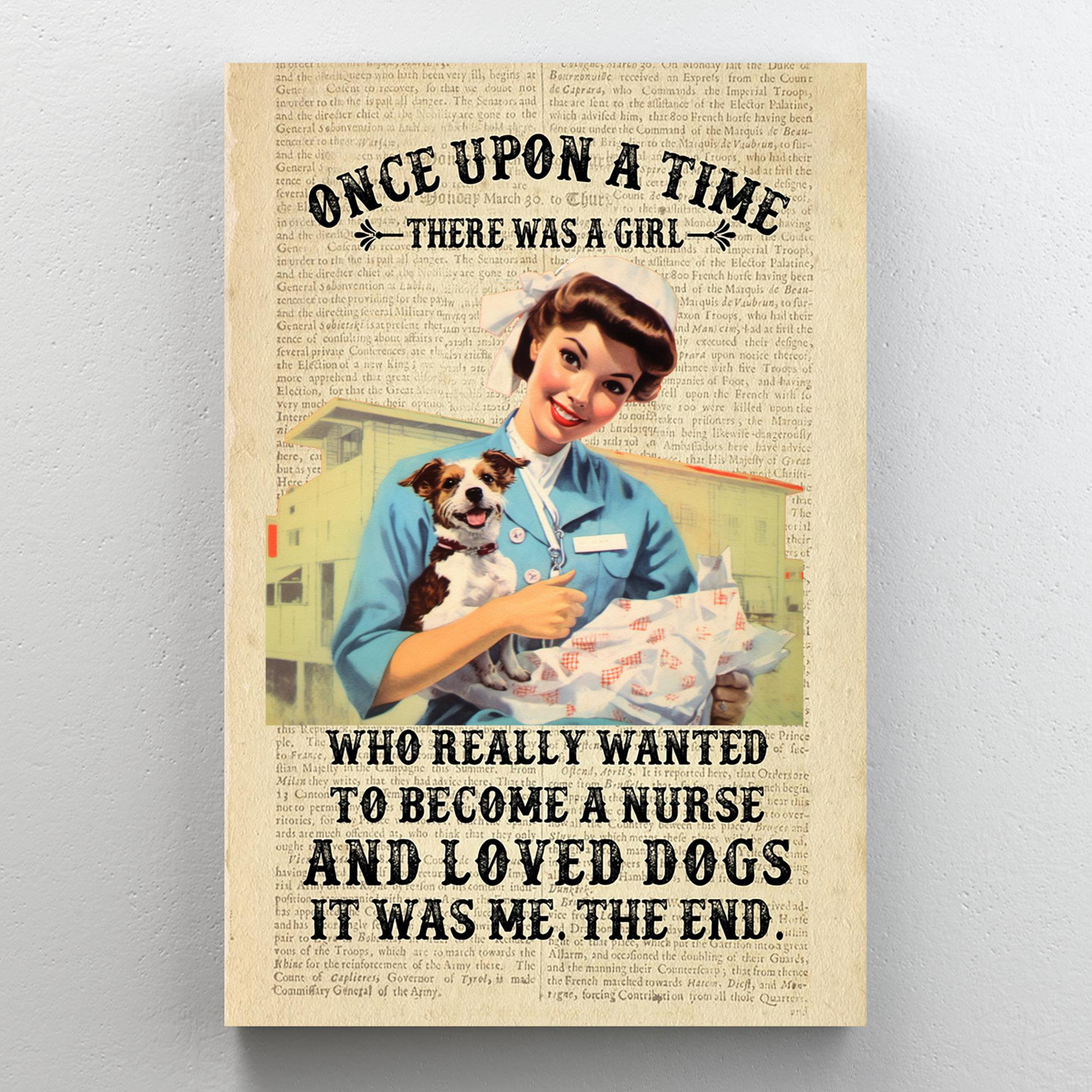The image depicts an old, yellowed book page with two columns of text that are too small to read. Overlaid on this page, there is a poster featuring a vintage illustration reminiscent of the 1950s. The top of the poster has a black, all-caps caption that reads, "ONCE UPON A TIME THERE WAS A GIRL." Beneath this text, there is a colored drawing of a young woman in her mid-twenties with brown hair styled in a white bandana. She is wearing a light blue nurse's coat and a white hat, with a stethoscope and a name tag visible. In her right arm, she cradles a small dog that appears to be a terrier. In her left hand, she holds a white tissue paper with red markings. A green building serves as the background. Below the illustration, the text continues: "WHO REALLY WANTED TO BECOME A NURSE AND LOVE DOGS. IT WAS ME. THE END." This amalgamation of a book page and poster creates a nostalgic and heartfelt portrayal of a young woman's aspirations and love for animals.